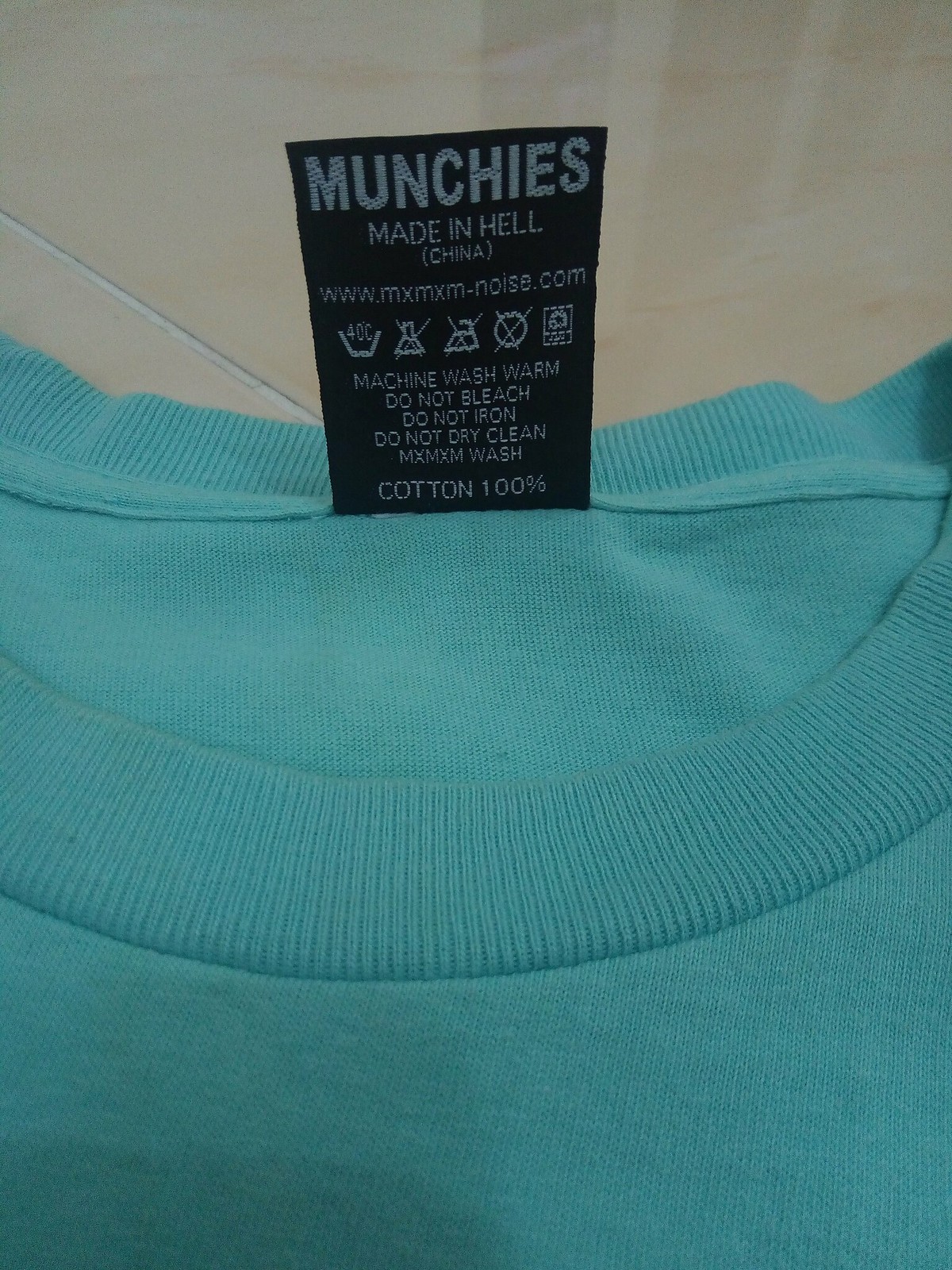This image features a close-up of the upper part of a turquoise round-neck t-shirt. The background consists of white tile, providing a stark contrast to the vibrant color of the shirt. The t-shirt's tag, which is square and flipped up, reveals the brand name "Munchies" boldly printed in white. Below the brand name, the tagline "Made in Hell" is written in all caps and enclosed in parentheses, followed by "China." The tag also includes a website address and detailed cleaning instructions.